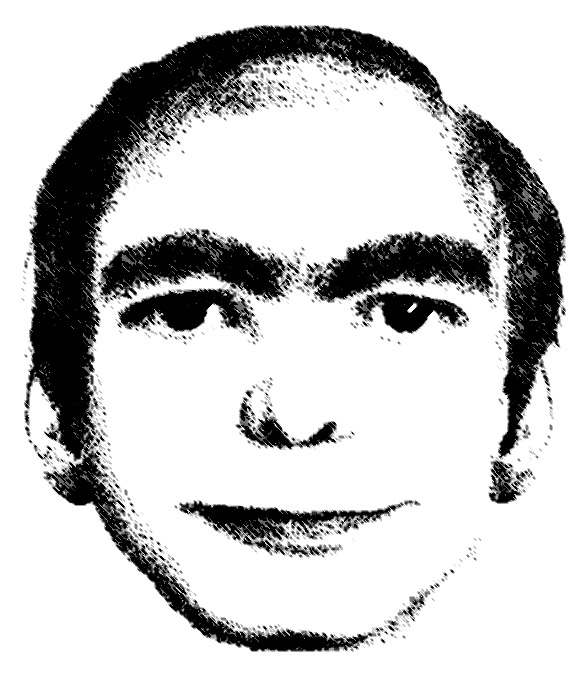This black-and-white photograph appears to be an old mugshot, focusing solely on the individual's face with no discernible background. The person captured in this image has a strikingly familiar appearance, reminiscent of a high-profile or infamous criminal from a bygone era. The most notable feature of the subject is his prominently thick, bushy, and dark eyebrows, which command immediate attention. He also has short black hair, which is receding slightly, adding to the overall aged look of the photograph. The person's expression is stoic, with sealed lips and a direct gaze into the camera, consistent with typical mugshot conventions. His nose is rounded, which is also a distinguishing characteristic. The photo, seemingly a cropped section of a larger piece, lacks color and additional context, focusing the viewer's attention on the distinguishing facial features that hint at a possible notorious past.